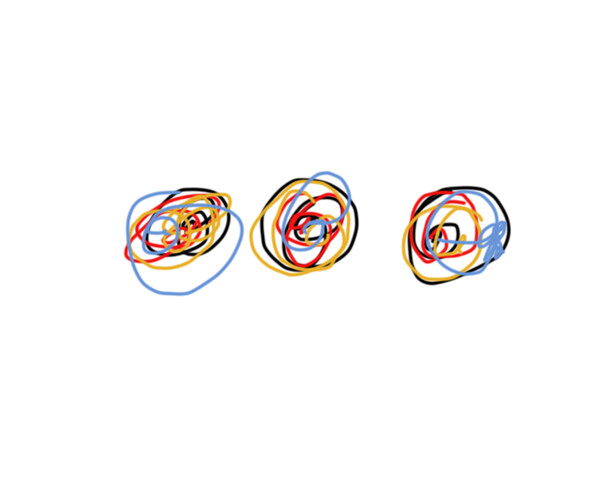This image showcases three intricate bunches of vibrant material that could either be colored string or rubber bands, arranged in circular loops interwoven with each other. Each cluster features a dynamic mix of light blue, black, golden yellow, and tomato red colors.

- In the far-left bunch, black and red hues form the backdrop while light blue and yellow strands dominate the foreground, creating a striking contrast.
- The middle group is characterized by the prominence of the tomato-red color, which stands out more than in the other two bunches.
- The far-right cluster is predominantly black and light blue, with the blue strands notably tied into a small knot or bow on the right side. This arrangement of blue and black creates a unique, textured appearance.

The overall composition is a complex network of squiggly lines that weave in and out of each other, some with visible loose ends, adding to the texture and depth of the image. The background is a pristine white, seamlessly merging into the webpage with no visible border, enhancing the focus on the colorful arrangements.